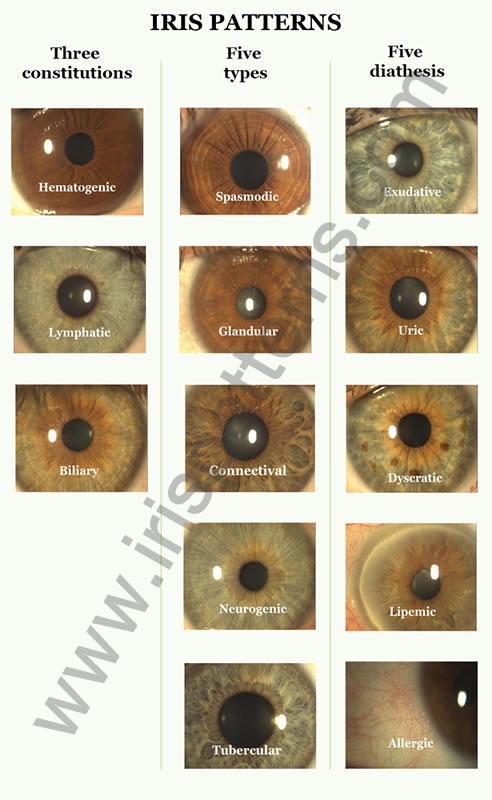The image is a detailed chart showcasing various human iris patterns, divided into three sections. At the top, bold black text reads "Iris Patterns." The sections are labeled as "Three Constitutions," "Five Types," and "Five Diatheses."

- **Three Constitutions**: This section features close-up photographs of eyes, labeled as Hematogenic, Lymphatic, and Biliary. Each photo displays a different color and pattern associated with its classification.
- **Five Types**: In the center, there are five distinct iris patterns, each named and displayed in individual boxes. The labels are Spasmodic, Glandular, Connectival, Neurogenic, and Tubercular.
- **Five Diatheses**: On the right, this column includes five rows, each showing an eye pattern associated with the categories Exudative, Uric, Dyscratic, Lipidemic, and Allergic. These images also illustrate various colors and conditions, with the Allergic one notably appearing bloodshot.

Additionally, there is a semi-transparent URL, www.iristerms.com, running diagonally from the bottom left to the top right corner of the image.